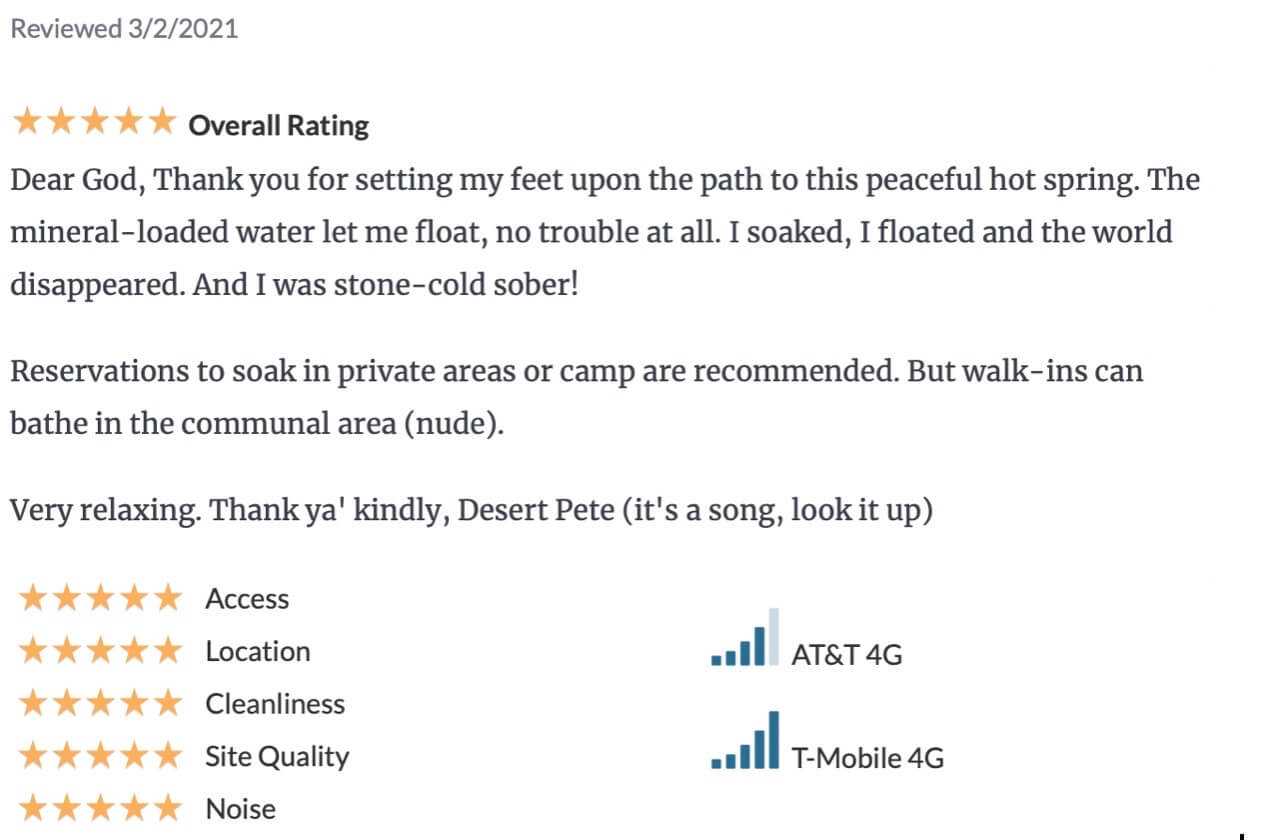### Detailed Caption:

This screenshot is presented on a white background with a gray font. At the top left, it is titled "Reviewed 3-2-2021." Adjacent to the title is a rating of five yellow stars, indicating a perfect score. Boldly marked next to it is the label "Overall Rating."

Beneath this label, the review reads: 

**"Dear God, Thank you for setting my feet upon the path to this peaceful hot spring. The mineral-loaded water let me float with no trouble at all. I soaked, I floated, and the world disappeared. I was stone-cold sober."**

Following this section, there's a recommendation regarding reservations: 

**"Reservations to soak in private areas or camp are recommended, but walk-ins can bathe in the communal area (nude)."**

Some blank space later, the review continues with a closing remark:

**"Very relaxing, thank you kindly. Desert Pea (it's a song, look it up)."**

Underneath, the review splits into categories, each with a corresponding five-star rating to the left:

1. **Access** - ☆☆☆☆☆
2. **Location** - ☆☆☆☆☆
3. **Cleanliness** - ☆☆☆☆☆
4. **Sight Quality** - ☆☆☆☆☆
5. **Noise** - ☆☆☆☆☆

On the right side of this section, there are two options displaying the phone service providers' coverage quality:

1. **AT&T 4G** - 4 out of 5 bars
2. **T-Mobile 4G** - 5 out of 5 bars

This part illustrates which provider has better reception at the location, indicating that T-Mobile has superior coverage with a full rating compared to AT&T.